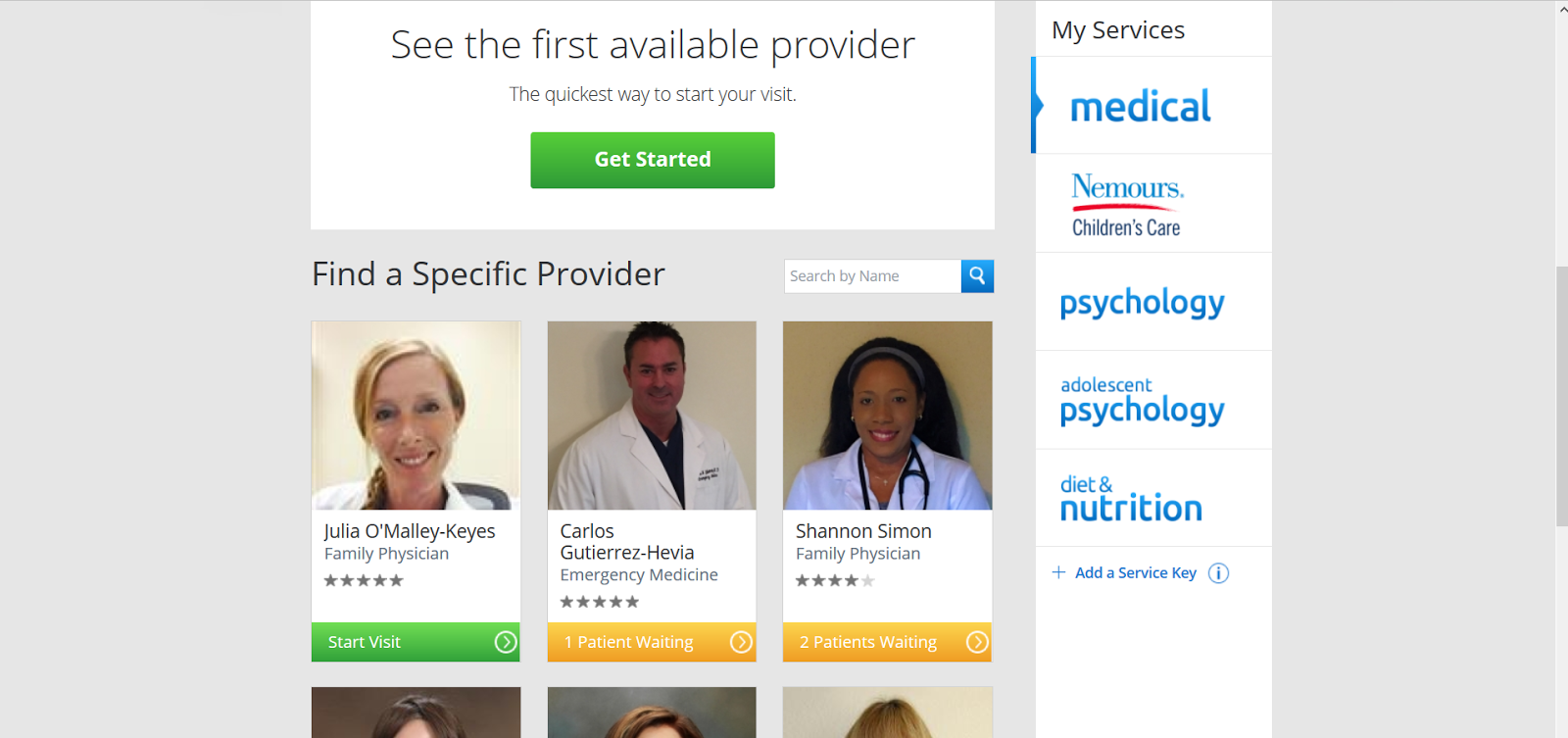Screenshot of a mobile app interface displaying a selection of healthcare providers. The screen is oriented horizontally with a predominantly gray background. In the center, there is a smaller rectangular section highlighting several doctors and their details.

At the top of this section, a heading reads, "See the first available provider: the quickest way to start your visit," followed by a prominent green "Get Started" button. Below this, there is an option to "Find a specific provider" with a search bar labeled "Search by name."

The main section showcases individual doctor profiles:
- On the left, Dr. Julia O'Malley Keyes, a family physician rated five stars, with a green "Start Visit" button beside her name.
- Beneath her, Dr. Carlos Gutierrez Hevia, an emergency medicine specialist, also rated five stars. His profile indicates "One patient waiting" in a yellow box. He is light-skinned with dark hair, wearing a white coat.
- To the right, Dr. Shannon Simon, a family physician rated four stars, has "Two patients waiting" in a yellow box. She is depicted as a black woman with long dark hair, smiling and wearing a white coat with a stethoscope around her neck.

Additionally, the tops of the heads of three more doctors can be seen at the bottom of the screen, suggesting more options are available if one scrolls down. On the far right side of the screen is a white bar listing services such as "Medical," "Children's Care," "Psychology," "Adolescent Psychology," and "Diet and Nutrition."